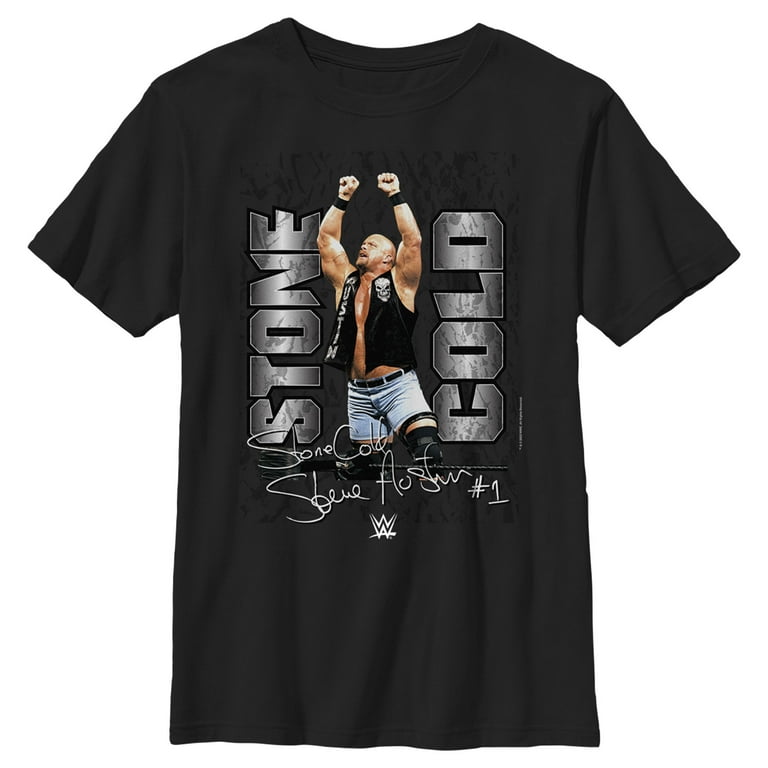This is a highly detailed, black t-shirt featuring the legendary wrestling superstar, Stone Cold Steve Austin. The t-shirt showcases a photorealistic image of Stone Cold in the center, a muscular, bald Caucasian man in his mid-40s with a goatee. In the image, he is standing triumphantly, presumably on the ropes of a wrestling ring, with both arms raised and fists clenched, his head tilted back as he yells in celebration.

Stone Cold is wearing black wristbands and a black sleeveless jacket. The right side of the jacket displays the word "Austin," while the left side features a white skull. He is clad in blue jean shorts with a black belt and has knee braces on both knees. The image on the t-shirt extends down to just above his knees.

Flanking the central image, the text "Stone" runs vertically on the left, and "Cold" runs vertically on the right. Below the image is a graphic of Stone Cold's signature, followed by the WWE insignia, cementing the t-shirt's authentic wrestling memorabilia status.